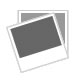This image depicts a hooded black cloak made from a shiny material, which appears short and likely to be worn over a longer garment. The cloak features a ribbon tie at the neck, and the hood is pointed. The backdrop is entirely white, and the cloak's dimensions are provided in black text: 45.5 centimeters at the top, 26 centimeters on the right, and 75.5 centimeters at the bottom. These measurements are accompanied by pink text showing additional dimensions - 40 centimeters at the top, 21 centimeters on the right, and 70 centimeters at the bottom. Asian characters, likely Japanese, are visible at the very bottom of the image. The cloak seems to be draped over an invisible form facing downwards to the left, creating an impression of it being worn yet empty.